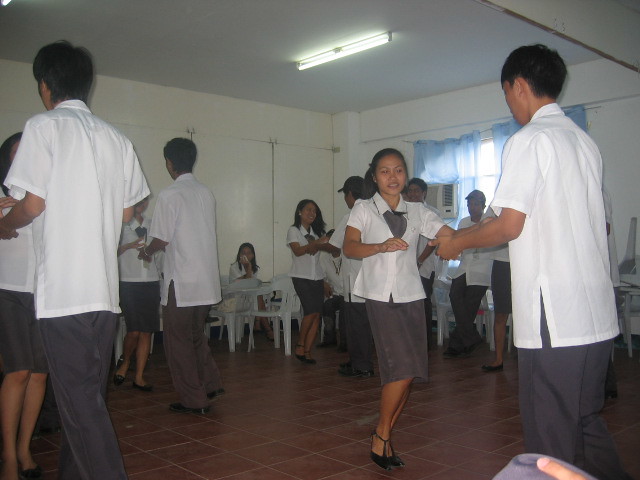In this image, a group of young Filipino teenagers in school uniforms is seen awkwardly learning to dance in what appears to be a gym class at a private school. The boys are dressed in white short-sleeved, button-down shirts with brown slacks and black shoes, while the girls wear similar white button-down shirts paired with brown skirts and a matching brown scarf around their necks. They are all paired off, holding hands with partners of the opposite gender, and appear to be enjoying the moment albeit somewhat self-consciously. The room features a brown tile floor, white walls, a white ceiling, and blue linen curtains hanging over the windows on the far right wall, which also houses an air conditioning unit. There are about ten students dancing, supervised by a couple of adults in similar attire. In the background, plastic seating lines one wall, with someone seated there.